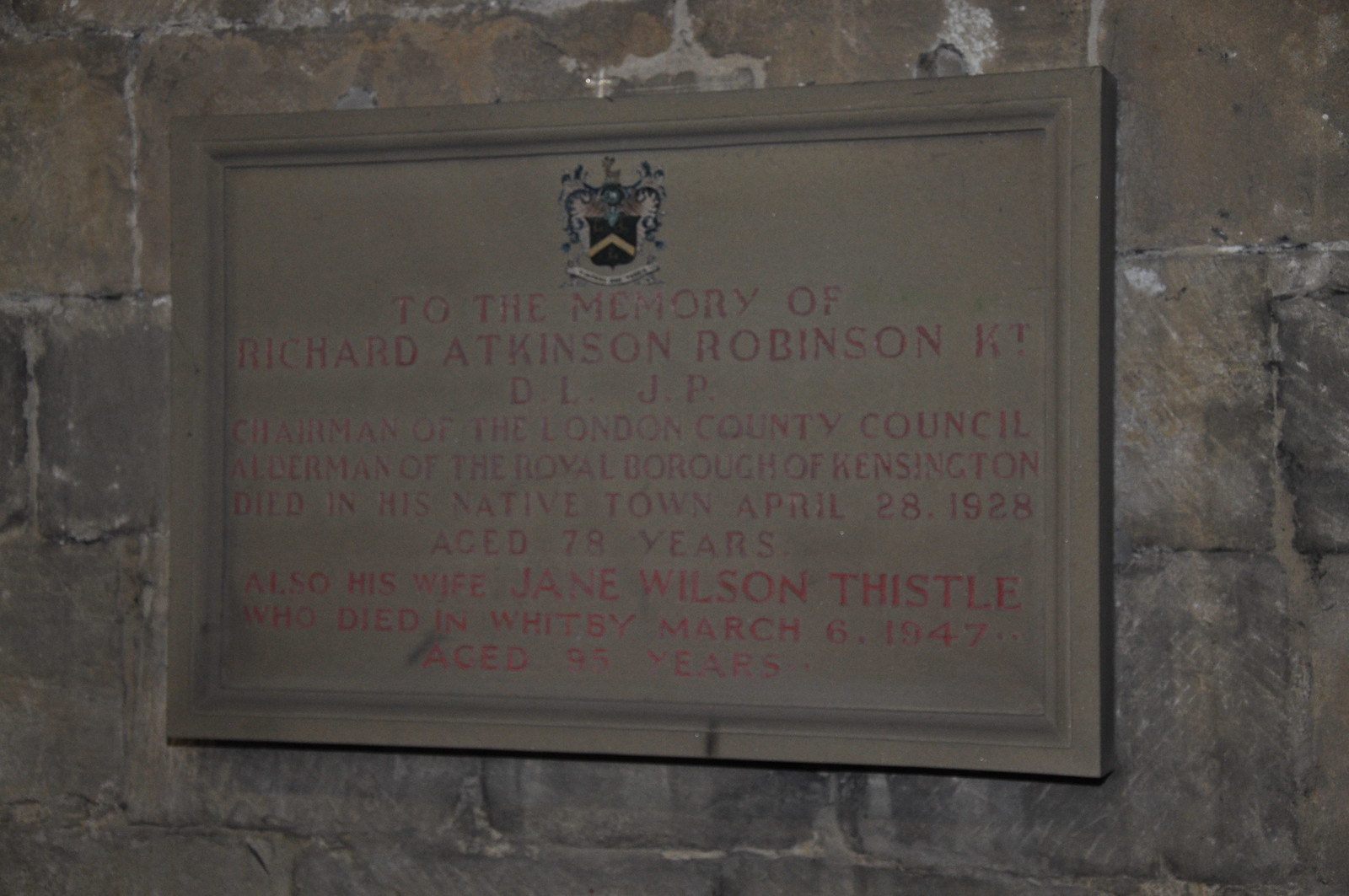This photograph features a weathered plaque mounted on a stone wall, possibly part of a tomb or monument. The plaque, framed in wood, bears dull, faded colors. At the top center is a majestic shield or crest. The text, though worn and difficult to read, is inscribed in uppercase red letters. It commemorates Richard Atkinson Robinson, bearing the initials K.T., D.L., J.P., noting his titles as Chairman of the London County Council and Alderman of the Royal Borough of Kensington. He passed away in his native town on April 28, 1928, at the age of 78. Beneath this, the plaque also honors his wife, Jane Wilson Thistle, who died in Whitby on March 6, 1947, at the age of 95.